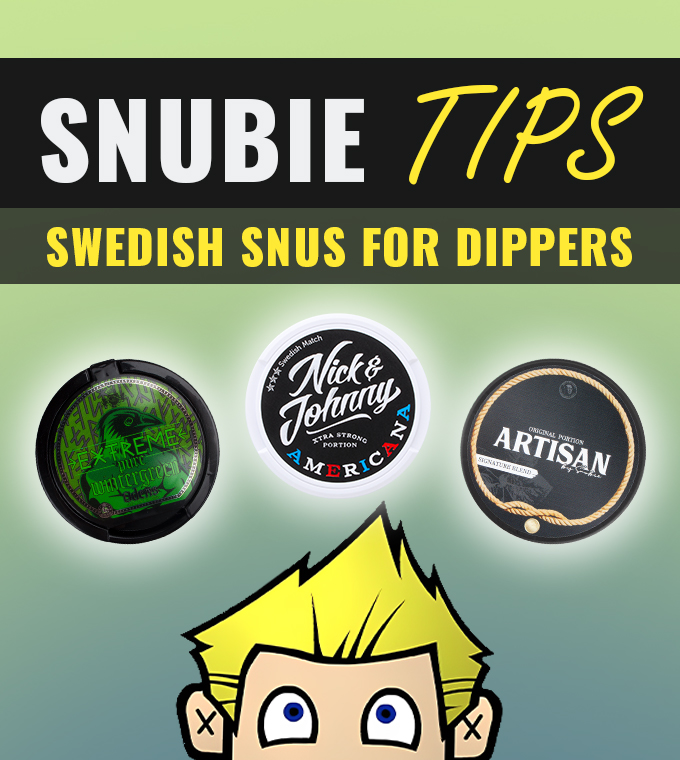The image appears to be a marketing advertisement for chewing tobacco, set against a light green background that fades into a darker greenish-blue at the bottom. At the top of the image, there's a black horizontal bar featuring bold white text that reads "SNUBIE" in all capital letters. To the right of this in yellow, handwritten print is the word "TIPS." Below this black bar is a gray horizontal bar with yellow, all-capital letters that read "SWEDISH SNUS FOR DIPPERS."

Beneath this section, there are three circular images arranged in an arc. The left circle is predominantly black with an inner green circle that features the word "EXTREME" in lighter green lettering across the center. The middle circle is also black, with script text that diagonally reads "NICK AND JOHNNY." Below this script, there is curved white text (too small to read) and additional curved text in red, white, and blue that spells "AMERICANA." The right circle features a black inner circle outlined in yellow and has horizontal white text that reads "ARTISAN." There is small, unreadable white text above and below the word "ARTISAN," with a white bar extending from the left of the circle containing more black print that is too small to decipher.

Below the arc of circles, there is a cartoon drawing of a blonde-haired man with hand-drawn facial features and eyes looking upwards. The man has blue eyes with exaggerated white circles for the eye whites and X's in his ears, giving a whimsical touch to the advertisement's overall design.